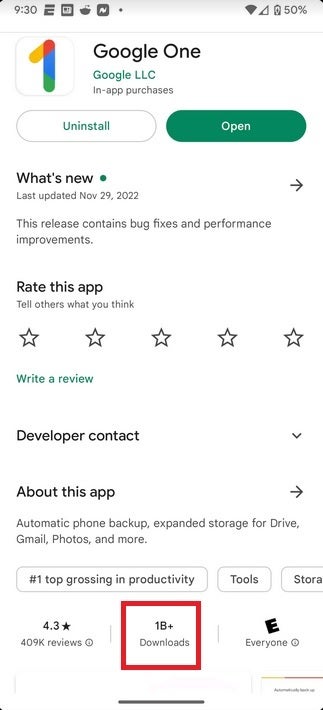This image appears to be a screenshot of a smartphone's screen, specifically from the Google Play Store. In the top-right corner, the status bar displays the time as 9:30, alongside icons for the Wi-Fi signal, cellular data signal, battery level at 50%, and app notifications including those from ESPN and Reddit. Below the status bar, the Google Play Store interface is clearly visible.

The focus of the screenshot is the Google One app page. At the top of this section, there is a banner with the Google One logo, followed by buttons for "Uninstall" and "Open," indicating that the app is already downloaded on the device. Beneath these buttons, it is noted that the app is developed by Google LLC and includes in-app purchases.

Further details on the page reveal the app's most recent update on November 29, 2022, with a brief description stating, "This release contains bug fixes and performance improvements." Users are invited to rate the app from one to five stars. Additional sections provide more information about the app's features such as automatic phone backup, expanded storage for Google Drive, Gmail, Photos, and more. The app holds the title of "#1 Top Grossing in Productivity Tool Storage."

The app's rating is prominently displayed as 4.3 stars, based on 409,000 reviews. It has over 1 billion downloads and is rated "E for Everyone," meaning there are no age restrictions for users.

In summary, this screenshot captures the Google One app page on the Google Play Store, showcasing details about the app, its functionality, user reviews, and download statistics.